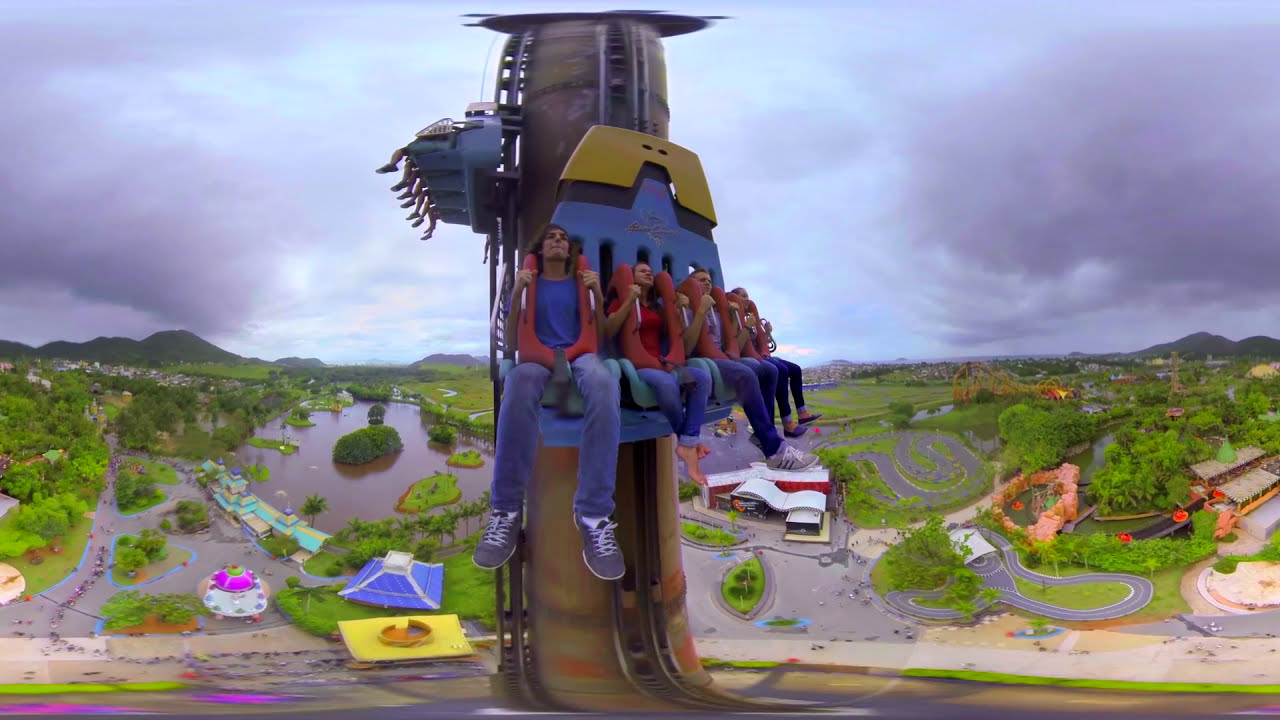This is a detailed shot of an amusement park, prominently featuring a towering drop tower ride. The ride, resembling a vertical column, is divided into three sections, each with five seats where riders are strapped in securely with over-the-shoulder restraints, their feet dangling freely. The photo captures the riders in a moment of anticipation or apprehension as they hold onto the handlebars around their chests at the peak of the ascent. The diverse park landscape unfolds behind them, including a vast lake or pond on the left, numerous rides such as roller coasters and go-kart tracks scattered throughout, various buildings and entertainment sections, tents possibly indicating food areas, and predominantly green expanses of trees and bushes. The background features a scenic horizon of mountainous regions under a cloudy sky with patches of blue, adding a dramatic contrast to the lively park beneath. The image is populated mostly by young Caucasian individuals and offers a vibrant mix of colors and structures set against a dynamic sky.